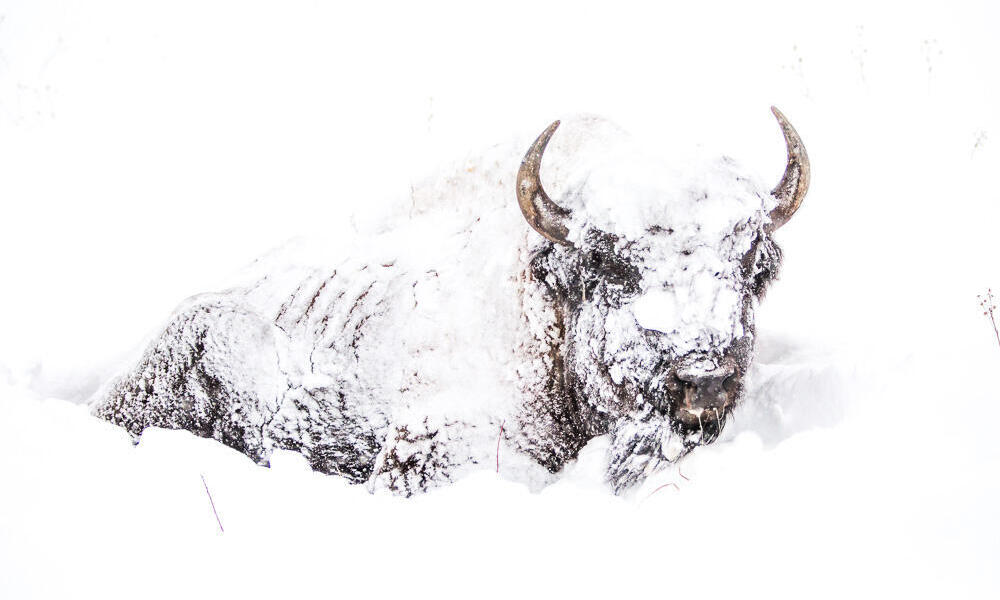This detailed drawing depicts a buffalo, its dark brown fur partially hidden beneath a thick layer of snow, giving the image a stark, almost monochromatic appearance. The buffalo's two prominent horns and faintly visible eyes and snout emerge through the dense snow, creating a striking contrast. Snow heavily coats the top of its head and the hump of its back, while areas around the flanks and neck showcase patches of exposed fur. The animal is positioned facing slightly forward and to the right, revealing an intricate balance between the white snow and the shaded details of its body. The drawing captures the essence of the buffalo almost fading into and out of the snow, with only the upper half visible, emphasizing its powerful presence amid a wintry, almost blown-out landscape.